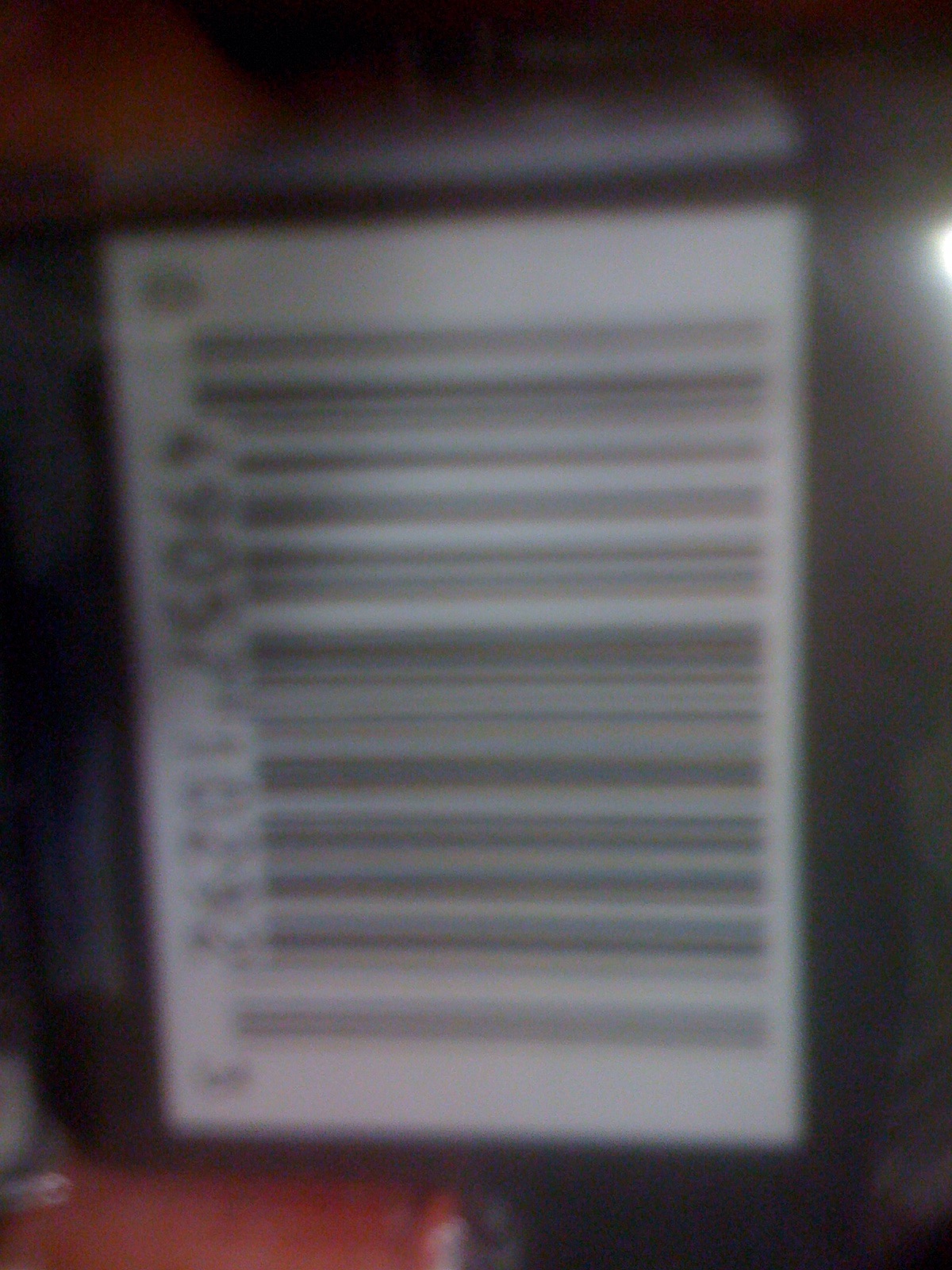This close-up photograph features a UPC code against a predominantly black and gray background. The image is notably blurred and hazy, which makes the subject less distinct. To the right of the frame, a bright light intrudes, adding to the overall lack of clarity. In the bottom left corner, a red surface is visible, contrasting with a minor tan area in the upper left. The positioning of the UPC code is tilted, with the vertical black lines and intervening white spaces running from top to bottom. The numbers of the barcode are challenging to discern due to the blurriness, but seem to read: 0 6 9 0 5 7 1 0 2 9 2 3.